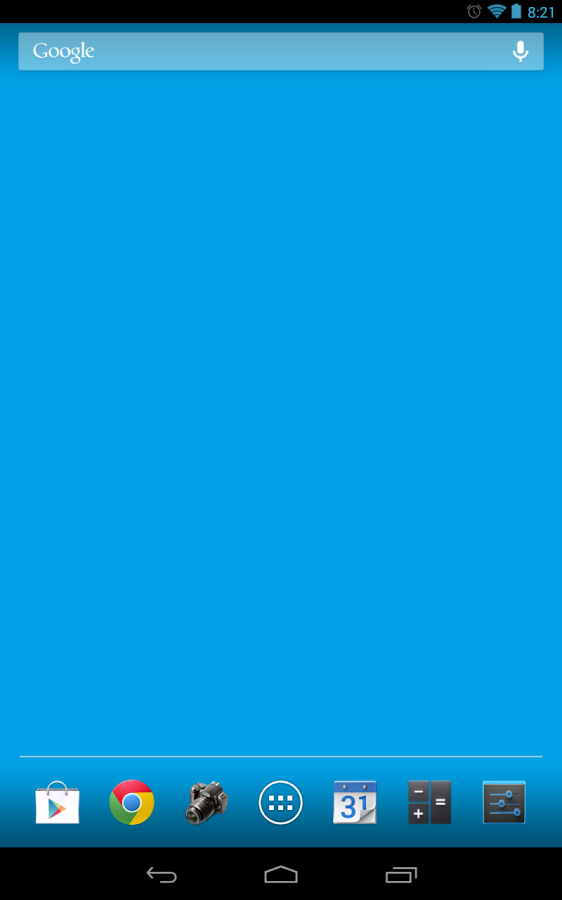This image showcases a screenshot of a cell phone home screen. 

- **Time and Status Icons**: In the upper right corner, the time is displayed as 8:21 with no AM or PM specification. Adjacent to the time, indicators show a full battery, a strong Wi-Fi signal, and an active alarm, represented by a small alarm clock icon.
  
- **Search Bar**: Below the status icons, a Google search bar spans the screen. On the right end of the search bar, there's a microphone icon for voice searches.

- **Background and App Icons**: The screen has a light blue background that extends down to the bottom of the display.

At the bottom portion of the screen:
  - **App Dock**: From left to right, the dock includes several icons:
    1. **Google Shopping**: An icon depicting a shopping bag with the Google logo.
    2. **Google Chrome**: The familiar Google Chrome browser icon.
    3. **Camera**: A black icon representing what appears to be a classic 35mm camera.
    4. **App Drawer**: A circle containing six white dots, symbolizing access to the app drawer.
    5. **Calendar**: An icon for the calendar app, showing the number "31" against a light blue background.
    6. **Calculator**: An icon with arithmetic symbols (plus, minus, equals), indicating a calculator app.
    7. **Equalizer/App**: A black icon featuring blue lines resembling an audio equalizer.

- **Navigation Bar**: At the very bottom of the screen, there are three navigation buttons:
  1. **Back Arrow**: On the left.
  2. **Home Button**: In the center.
  3. **Multitasking**: An icon of multiple boxes for toggling through open apps, positioned on the right.

The detailed layout and iconography reflect a typical modern Android smartphone home screen, outfitted with essential apps and utilities for daily use.